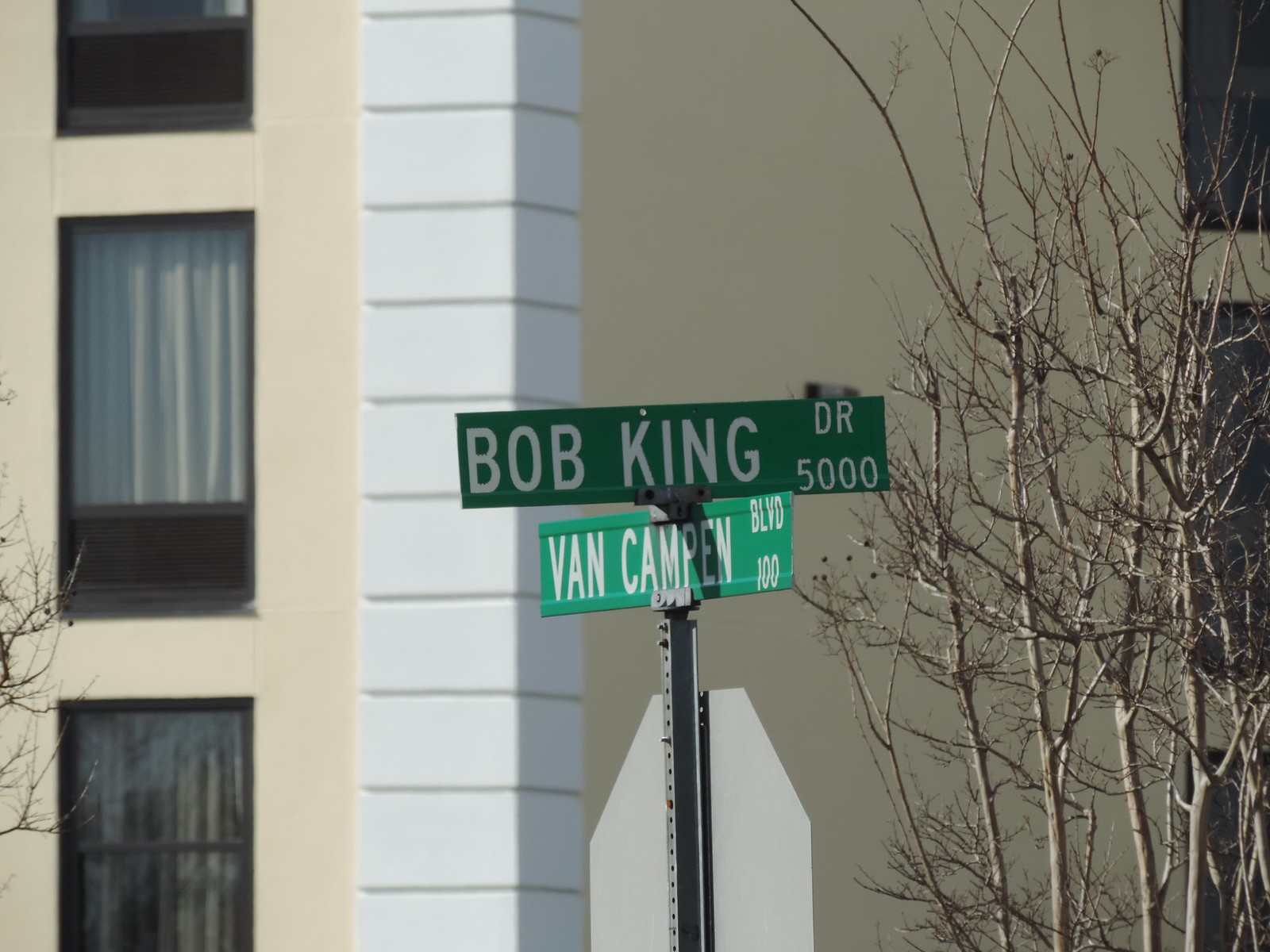This colour photograph captures a street sign pole positioned in front of a substantial apartment building devoid of leaves. The signs, typical of American street indicators, feature familiar green backgrounds with white text. At the top, a sign reading "Bob King DR" with the number "5000" directly below faces the camera. Perpendicular to it, the lower sign reads "Van Kampen BLVD" and displays the number "100." The metal pole hosting the signs has vertical perforations. In the backdrop, an expansive beige stone building with smooth stucco finish and horizontal white blocks on the corner dominates the scene. Visible are several windows with black frames and white curtains. Adjacent to the pole, a branchy, leafless tree extends into the frame, adding a stark contrast to the urban setting. At the bottom of the pole, the back of an octagon-shaped sign, presumably a stop sign, is visible, contributing an additional urban element to the detailed cityscape.